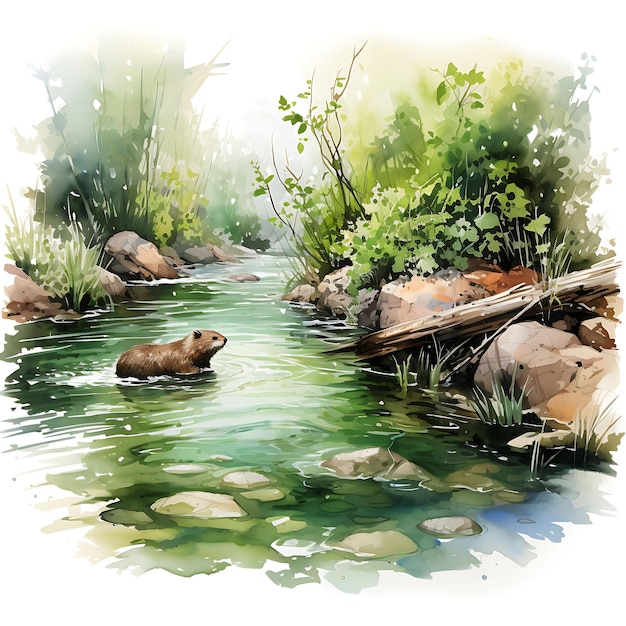This detailed watercolor painting captures a serene nature scene featuring a shallow, rippling stream that flows towards the viewer, framed by dense foliage with varying green hues and various vegetation types, including tall, lanky plants and bushes with green leaves. A beaver, positioned in the center-left of the painting, facing right, adds focal interest to the image. The beaver is depicted in the water, surrounded by scattered rocks, both in and along the banks of the stream. The water appears greenish and smooth, with visible rocks beneath its shallow surface. A fallen log slants upwards to the left, and the entire scene is rendered in muted greens, browns, and tans, fading into indistinct edges within a circular frame, which emphasizes the natural, tranquil setting. The background features hazy, indistinct details that add depth to the painting.